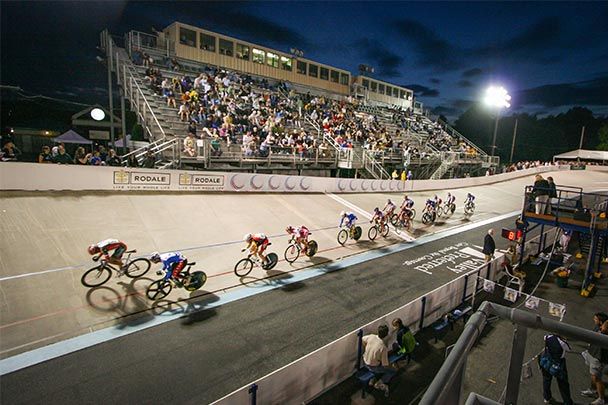The image depicts a nighttime bicycle race taking place in an outdoor stadium. The sky above, predominantly navy blue with some gray clouds, hints at nightfall, though the stadium is brightly illuminated by powerful floodlights. The racetrack, which has a slight curve to it, is surrounded by various elements contributing to the lively atmosphere of the event. 

On the track, you see more than a dozen cyclists in different uniforms, spread out in various positions—some at the front, middle, and rear of the race. The track itself features a white or beige surface with a green strip along its edge. To the right side of the image, beyond the barrier marked with the inscription "Rodale," spectators are visible; some are standing behind the border, while others are seated in bleachers, intently watching the race unfold. Additionally, there is a platform with steps leading up to it, where a stand seemingly designated for judges or announcers is stationed. The various perspectives and elements capture the energetic essence of the bicycle race within this well-lit nighttime stadium.